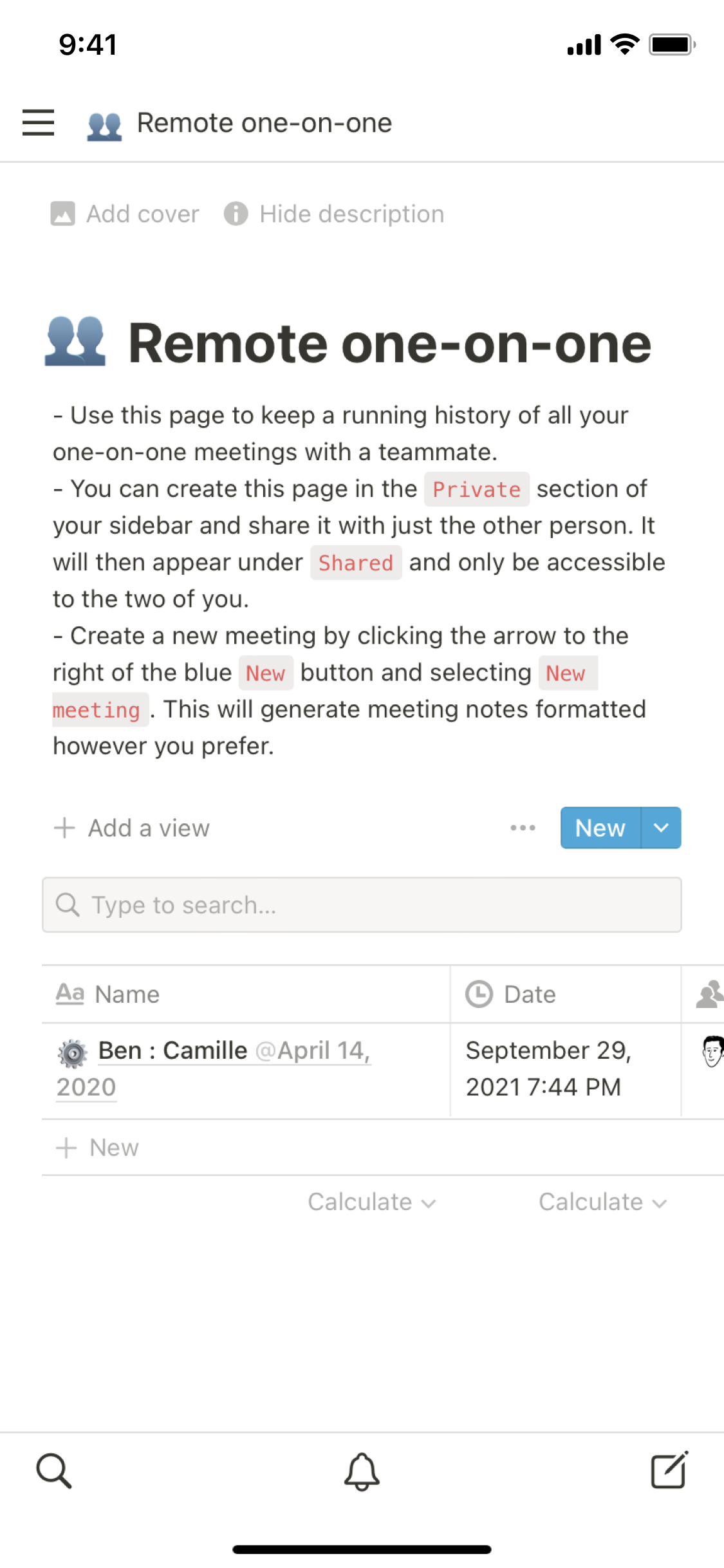The image showcases a smartphone screen with various icons and text. 

At the top right corner, there's a fully charged battery icon. Adjacent to it on the left are a Wi-Fi icon and a signal strength indicator, both showing full bars. In the top center, the title "Remote One-on-One" is displayed. Below this title, two buttons are visible: "Add Cover," which is accompanied by a small square portrait-like icon, and "Hide Description," next to a circular icon with an eye.

Prominently in the middle of the screen, "Remote One-on-One" appears again in larger black text. Underneath, an instructional sentence reads: "Use this page to keep a running history of all your one-on-one meetings with a teammate. You can create this page in the private section of your sidebar and share it with just one other person." The word "private" stands out in red against a gray background.

Towards the bottom of the screen, three icons are lined up: a magnifying glass on the far left, a bell in the center, and a square with a pencil on the far right. Above these icons, there's a section labeled "Name and Date," with the date specified as September 29th.